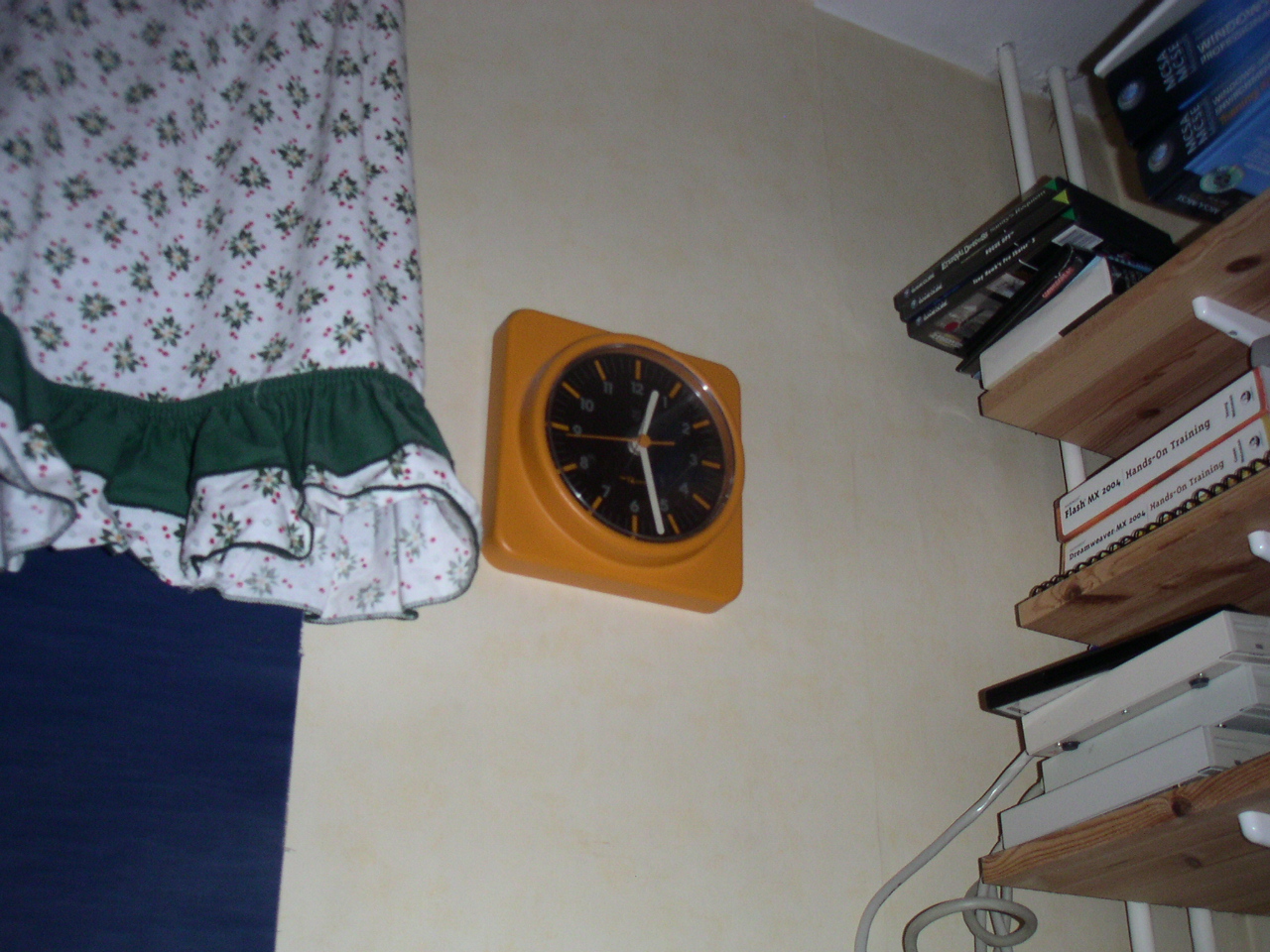This image captures the interior of a room, predominantly highlighting a beige wall adorned with an orange clock. The clock is square with a circular section that houses its black face. Orange lines mark the hours, with white numerals from 1 to 12 – though they are barely visible. The clock shows the time as 12:27, with white hour and minute hands, and an orange second hand.

To the right of the clock is a three-tiered wooden shelf system supported by white brackets. These shelves are filled with books, mostly positioned with the pages facing outwards, hiding the spines. On the middle shelf, two books are stacked, with visible text reading "Made" and "Hands on Chaney," though other details remain unreadable. The top shelf holds items that appear to be books or possibly software cases. 

Two poles extend from the shelf system to the ceiling, suggesting this might be a basement. To the left of the clock are old-fashioned curtains, predominantly white with a pattern of small green splashes and red dots, then finished with a green skirt and trim. A hint of something blue can be seen behind the curtains, adding another layer to the room's quaint and charming decor.